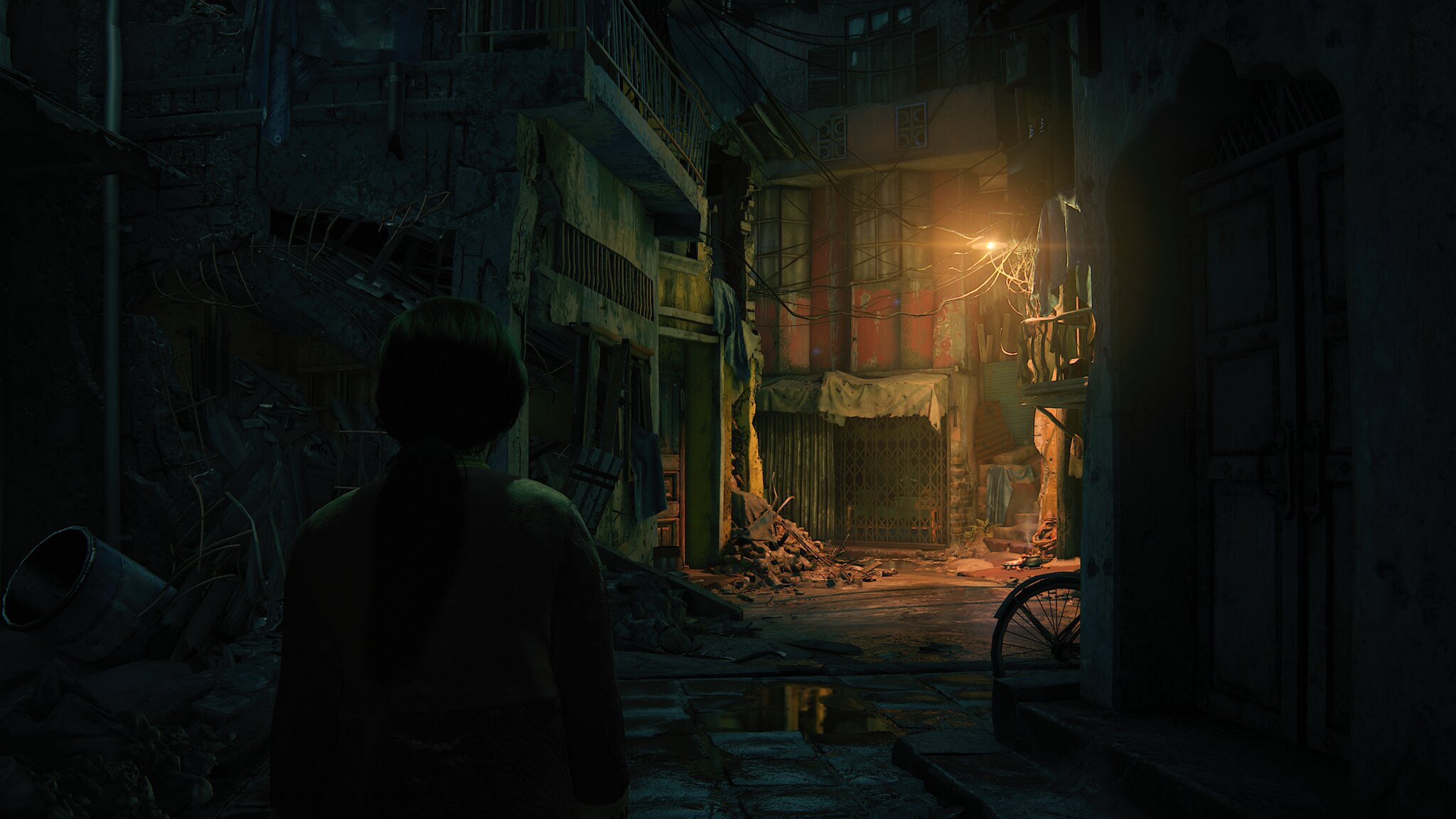In this stark and shadowy image, reminiscent of a scene from an animated movie or video game, we see the back of a person standing in a dimly lit, decrepit alleyway. The predominant palette consists of dark blues, reds, oranges, yellows, and hints of turquoise, creating a somber atmosphere. The alleyway is flanked by dilapidated buildings, some with busted windows and boarded-up entrances. Debris, including bricks and other materials, litter the ground, emphasizing the rundown state of the setting. To the left, trash is strewn about, and to the right, a bicycle wheel juts out from behind one of the structures. Overhead, telephone wires criss-cross the space. A solitary street lamp provides the only illumination, casting eerie shadows across the scene. The person, wearing a jacket, stands with their back to the viewer, their hair reaching down to the nape of their neck, adding a solitary human element to this otherwise desolate urban fragment.